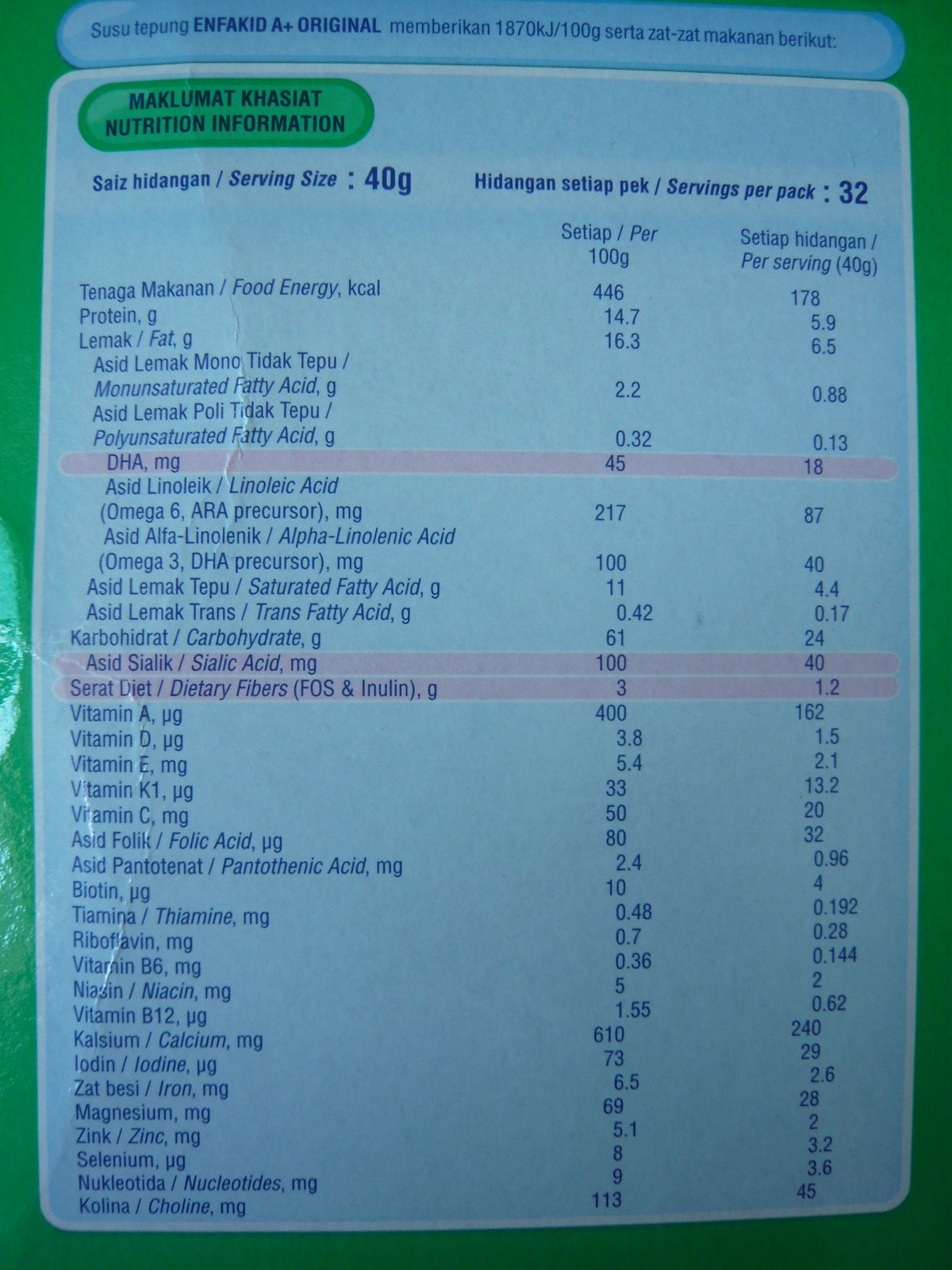**Product Name: Maclamat Kaziat Nutrition Information**

This detailed nutrition label appears to be from a foreign country and contains information for a product called "Maclamat Kaziat." The serving size is 40 grams, with a total of 32 servings per pack.

- **Calories**: 446 kcal
- **Protein**: 14.7 grams
- **Fat**: 16.3 grams
  - **Monounsaturated Fat**: 2.2 grams
  - **Polyunsaturated Fat**: 0.32 grams
- **DHA**: 45 milligrams
- **Omega Fatty Acids**: 217 milligrams
- **Saturated Fatty Acids**: 11 grams
- **Trans Fatty Acids**: 0.42 grams
- **Carbohydrates**: 61 grams
  - **Dietary Fiber**: 3 grams
- **Sialic Acid**: 100 milligrams
- **Vitamins**:
  - **Vitamin A**: 400 grams
  - **Vitamin D**: 3.8 grams
  - **Vitamin E**: 5.4 grams
  - **Vitamin K1**: 33 grams
  - **Vitamin C**: 80 grams
  - **Pantothenic Acid**: 2.4 grams
  - **Biotin**: 10 milligrams
  - **Thiamine (Vitamin B1)**: 0.48 milligrams
  - **Vitamin B6**: 0.36 milligrams
  - **Vitamin B12**: 1.55 milligrams

- **Minerals**:
  - **Calcium**: 73 milligrams
  - **Iodine**: 6.5 micrograms
  - **Magnesium**: 69 milligrams
  - **Zinc**: 8 milligrams
  - **Selenium**: 9 micrograms
  - **Choline**: 113 milligrams

This meticulously detailed label provides comprehensive nutritional information for consumers, including essential vitamins, minerals, fatty acids, and other nutritional components.